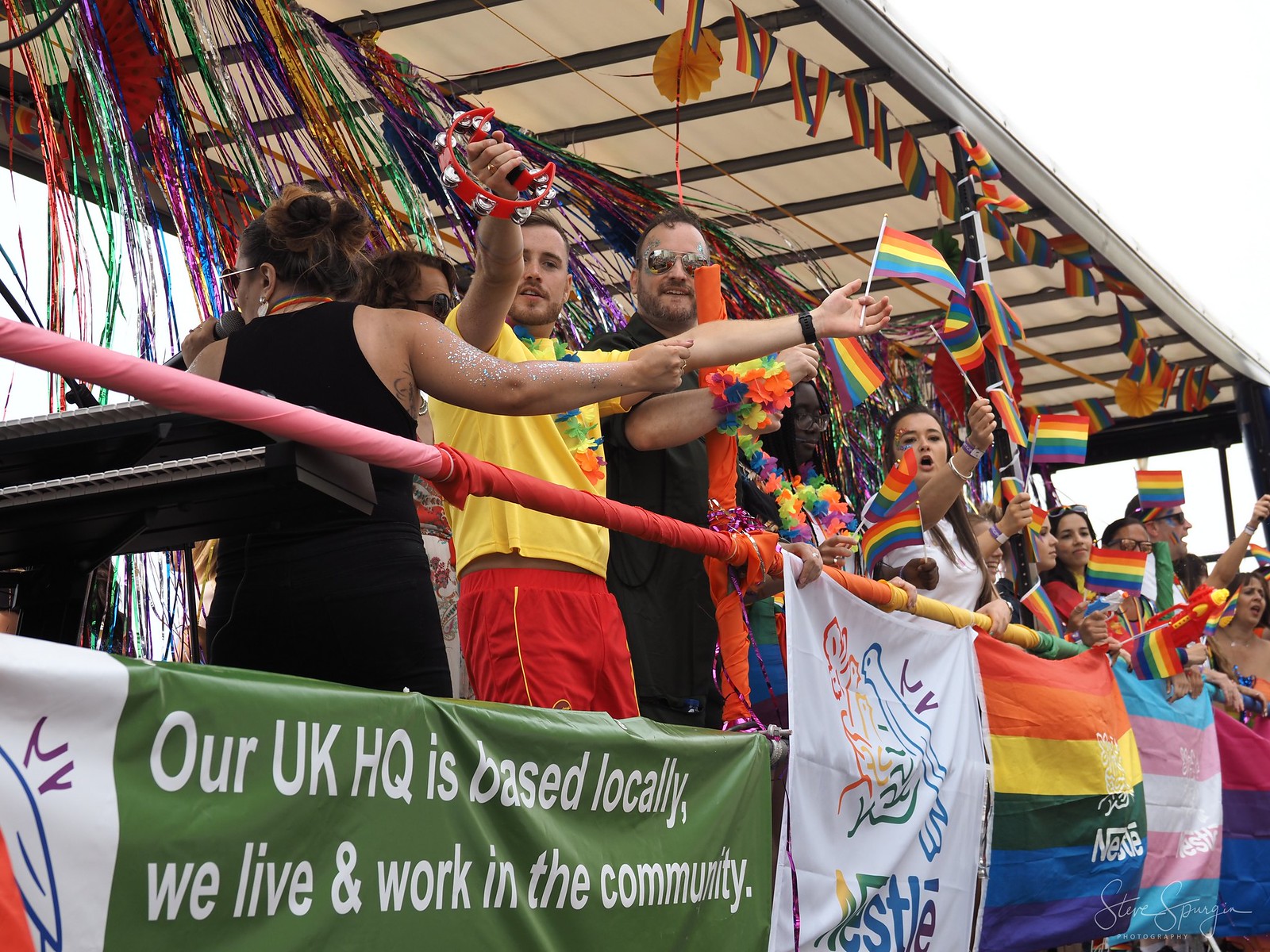In this photograph taken outdoors, several people are standing on a festive parade float, adorned with an array of colorful elements celebrating LGBTQ pride. The float features a large overhang from which streams of rainbow-colored strings are hanging, creating a vibrant canopy. At the center of the scene, a man in a yellow shirt and white shorts energetically waves a tiny rainbow flag; he also holds a tambourine, adding to the celebratory atmosphere. He is flanked by a man wearing sunglasses and a black shirt, who is also adorned with rainbow paraphernalia.

As your eyes travel along the float, you notice multiple pride flags being waved by individuals, contributing to the exuberant display. The side of the float prominently features several banners. One green banner with white font declares, "Our UK HQ is based locally. We live and work in the community." Adjacent to it is another rainbow-colored banner that reads "Nestle," melded into the vibrant background of various pride flags.

A piano is visible on the far left, further emphasizing the musical and festive setting. The backdrop of the float is predominantly white, enhancing the brilliant colors of the flags and banners. The people aboard are inside an enclosed section of the float, adding a layer of intimacy and togetherness to the joyous celebration. The scene is a rich tapestry of colors and symbols representing the diverse factions within the LGBTQ community.